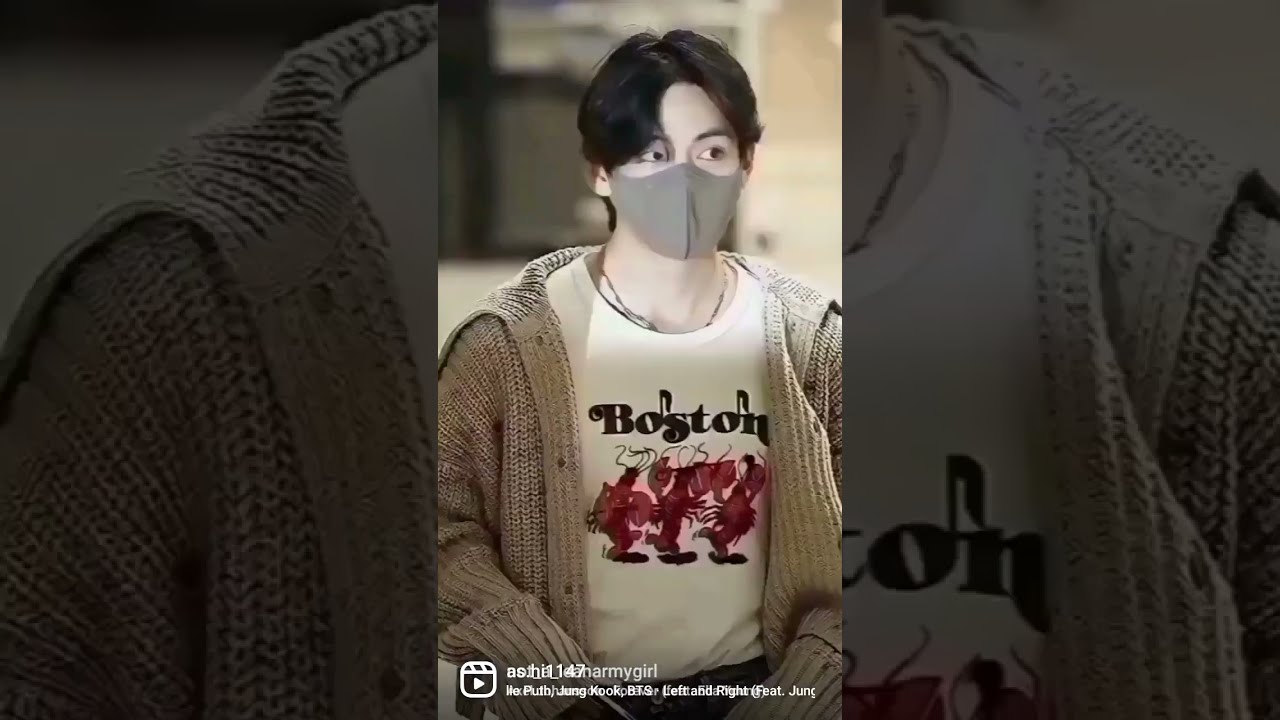The image features a young Asian male with black, center-parted hair, wearing a gray mask reminiscent of those used during the coronavirus pandemic. He is clad in a brown knitted sweater over a white t-shirt emblazoned with "Boston" and an image of what appears to be dancing crabs or lobsters. The subject appears to be seated, possibly with his arms crossed over his legs, and is positioned in a well-lit area with a blurred background. The photograph in the center panel occupies the majority of the composition, approximately 75-80%, while the left and right panels are zoomed-in, darker sections of the same image, creating a dramatic effect. At the bottom of the image, there are overlapping watermarks and text that are too small and blurred to be legible, possibly indicating an Instagram post with music tagging or other details. The overall composition and the person's appearance suggest a polished and styled presentation, possibly hinting at a K-pop star or influencer.